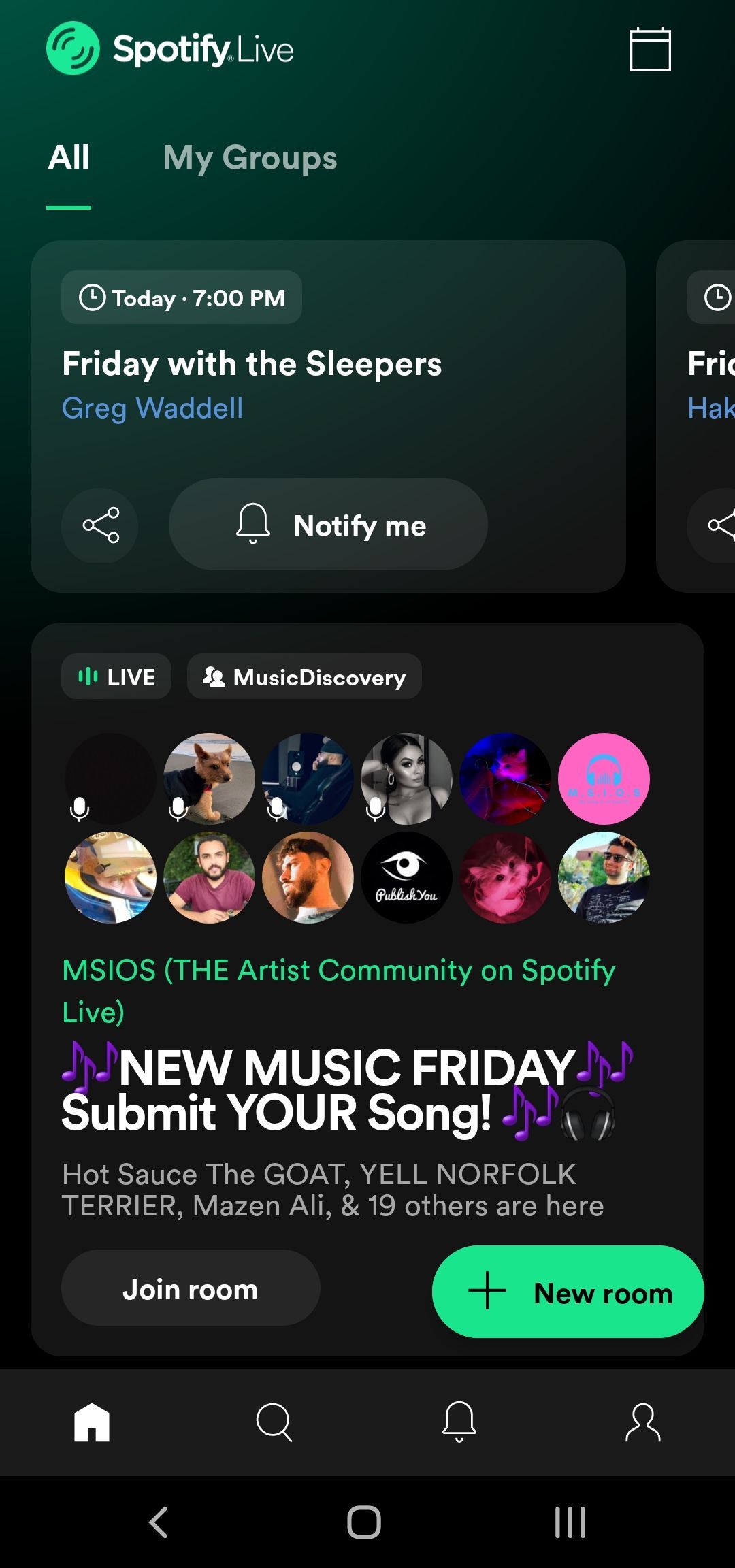The image features a black background primarily showcasing the Spotify Live interface. 

At the top, there's a green circle with black lines emblazoned with the text "Spotify Live." To its right, a small calendar icon is visible. Below, the section title "My Groups" is prominently underlined in green.

Directly underneath, a black box displays an event scheduled for "Today at 7:00 p.m., Friday" titled "The Sleepers." The name "Greg Waddell" is highlighted in purple, with a sideways 'V' icon next to a "Notify Me" button.

A subsequent black box features a series of approximately 11 circular profile images, including those of a dog, a lady, a pink icon with headphones, a guy, a cat, another dog, another guy, a guy at a desk, and a blue image, among others. This section is labeled "MSIOS The Artist Community on Spotify Live" in green text.

Adjacent are purple musical notes with the prompt "New Music Friday: Submit Your Song," along with additional sets of musical notes and a small headphones icon.

Following this, several usernames are listed: Hot Sauce, The Goat, Yale, North Folk, Terrier, Maison Alley, and 19 others, indicating that these users are present. A green "Join Room" button and a green plus symbol labeled "New Room" are presented as call-to-actions.

At the bottom of the image are navigation icons, including "Home," a magnifying glass for search, a bell for notifications, and a person icon. The very bottom features a left arrow within a square icon.